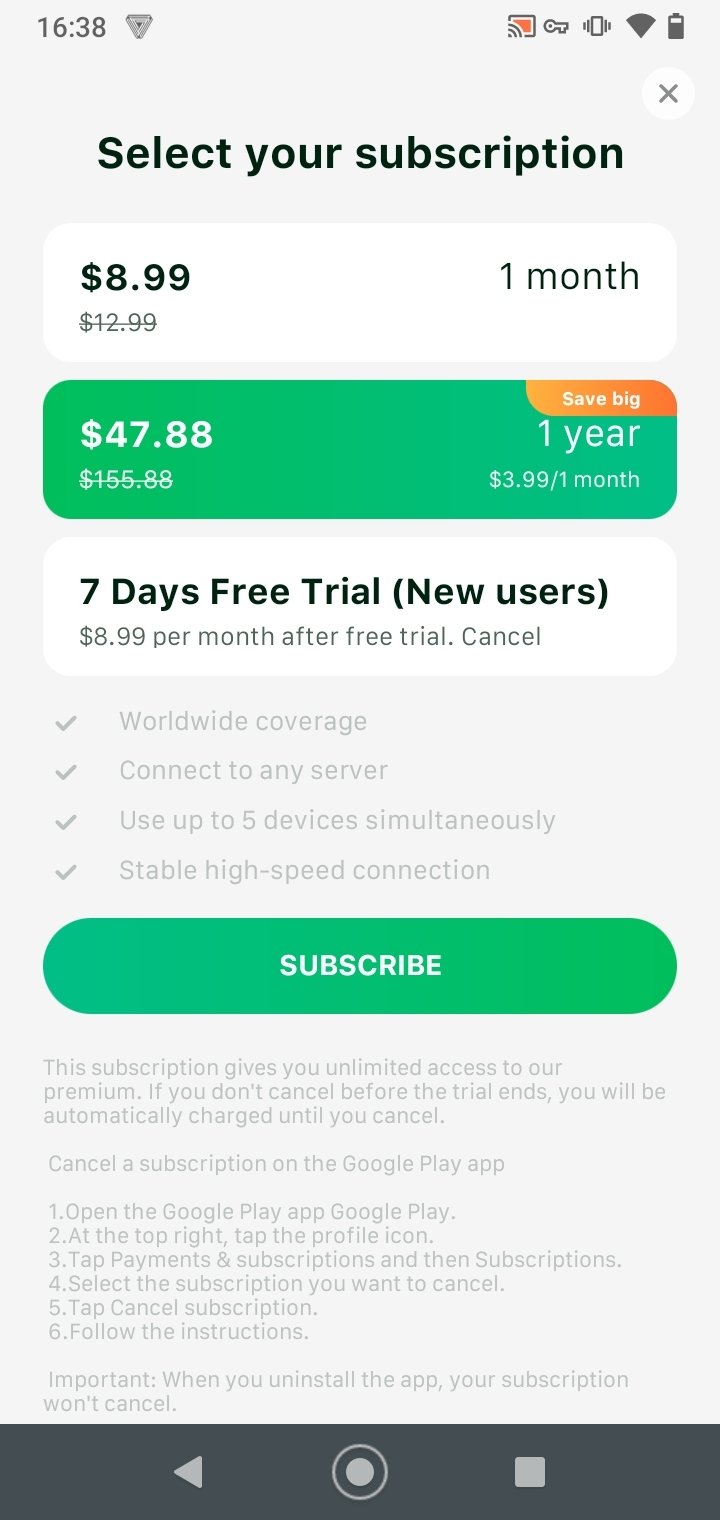**Detailed Image Caption:**

The screenshot is captured from an Android mobile device, identifiable by the navigation buttons at the bottom comprising a left-facing arrow for back, a circular home button, and a square button for accessing recent apps. The screen displays a subscription selection interface, likely from a browser page or an in-app page dedicated to subscribing to a service. 

At the top of the interface, there is a call to action with the text "Select Your Subscription" in bold black letters, accompanied by a close button represented by a white circle with an 'X' inside, allowing the user to exit the page.

Three subscription options are presented below this heading:
1. The first option features a white box indicating a price of $8.99 for one month, a reduction from the original price of $12.99.
2. The highlighted and likely selected second option is detailed within a green box. It offers an annual subscription at a discounted rate of $47.88, down from $155.88, which breaks down to approximately $3.99 per month.
3. The third option is for new users, offering a seven-day free trial, after which the service costs $8.99 per month.

The interface concludes with a green "Subscribe" button, inviting the user to confirm their subscription choice. The page is designed for clarity and highlights the most cost-effective subscription visually to draw the user's attention.